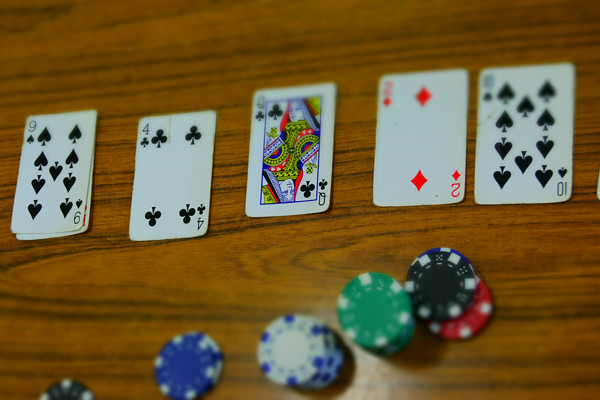In the photograph, we observe a rectangular landscape featuring a wooden table with a medium brown finish, the darker grains running horizontally from left to right, polished to a smooth sheen. At the center of the image, we find five playing cards laid face up in an informal arrangement. From left to right, the cards displayed are: the nine of spades, the four of clubs, the queen of clubs, the two of diamonds, and the ten of spades. The two of diamonds and the ten of spades are positioned closer together compared to the other cards, while the four of clubs sits slightly lower in the row. The angle of the cards is such that they tilt slightly to the left. Beneath the nine of spades, a partially obscured red playing card peeks out, with only about 5% of its full design visible.

At the bottom of the image, various stacks of poker chips are distributed. In the lower left corner, a black poker chip with white squares around the edge is halved by the frame. To its right, under the four of clubs, two blue poker chips are stacked. Further right, below and distant from the queen of clubs, four white poker chips with blue squares around the edges are seen in a stack. Continuing rightward, two more stacks appear: one green with white rectangles around the edge and one multicolored. The latter stack consists of three chips—a red one at the bottom, a blue one in the middle, and a black one on top, slightly offset from each other. These two stacks are positioned beneath the two of diamonds and ten of spades. The arrangement of these chips adds depth and color contrast to the composition.